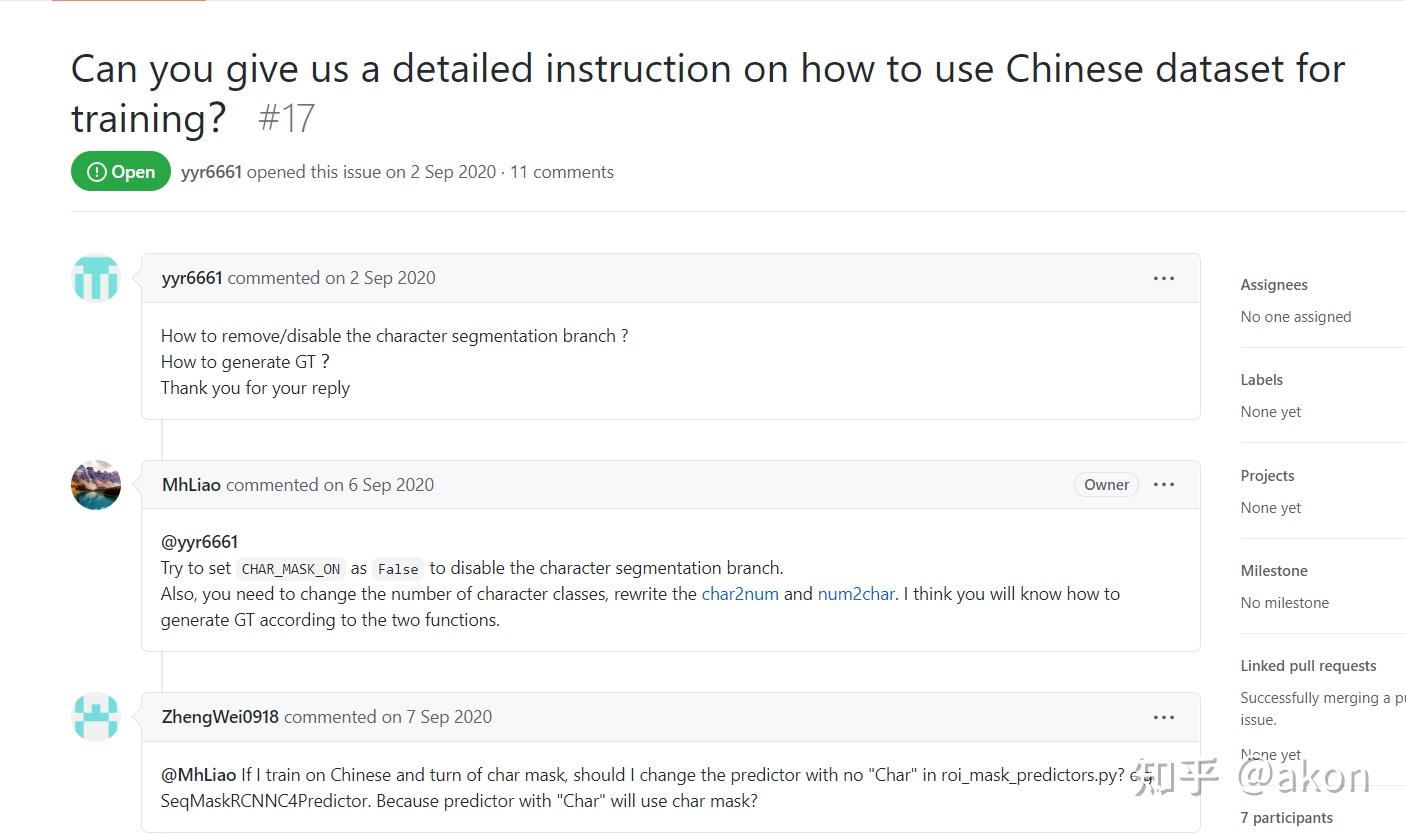**Caption:**

A screenshot of a web forum post detailing a discussion on how to use a Chinese dataset for training a machine learning model. The post is displayed on a clean, white background with black text. The initial question, posted by user YYR6661 on September 2, 2020, and labeled as Issue #17, asks for detailed instructions on using a Chinese dataset for training. The post remains open and has garnered 11 comments.

The first comment inquires about disabling the character segmentation branch and generating ground truth (GT). User M.H. Lyle responds, advising to set the `CHAR_MASK_ON` parameter to false to disable the segmentation branch and modify the number of character classes. They also mention the need to rewrite character and number functions, implying that the user will understand how to generate GT from these adjustments.

Another user comments, asking if they should modify the predictor to `NO_CHAR_ON_ROI_MASK_PREDICTORS` when training on Chinese with the character mask turned off, as the predictor with `CHAR` will use the character mask. The discussion reflects an ongoing attempt to adapt the training processes for a Chinese dataset effectively.